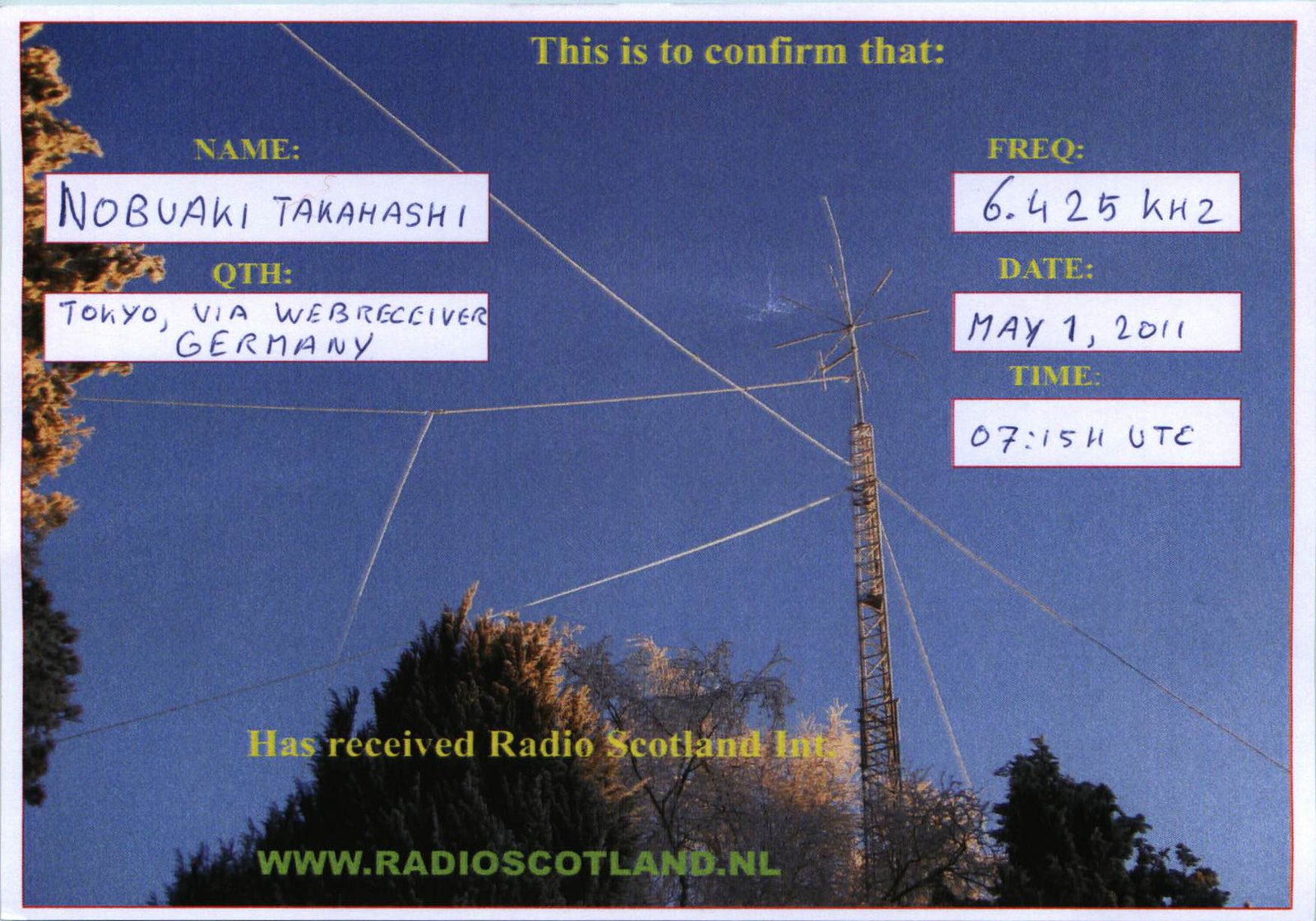This outdoor image, taken as a digital screenshot of a confirmation pass, is dominated by natural and man-made elements. The top of the pass features the text "This is to confirm that" followed by placeholders for name, date, and time. The image contains spaces for detailed information: "Name: Nobuaki Takahashi," "QTH: Tokyo," "DOF: Receiver Germany," "Frequency: 6.425 kilohertz," "Date: May 1st, 2011," and "Time: 7:15 HUTC." The confirmation message, in yellow print, states that it has received "Radio Scotland International," with the website "radioscotland.nl" also displayed in green. The background showcases a vivid green sky, possibly indicating a fall season due to the somewhat lifeless appearance of nearby trees. Prominent in the image are metallic structures resembling a radio tower with attached cables. The stark contrast of colors—blue, white, gray, black, and green—highlights both the natural scenery and the industrial elements of the radio equipment.